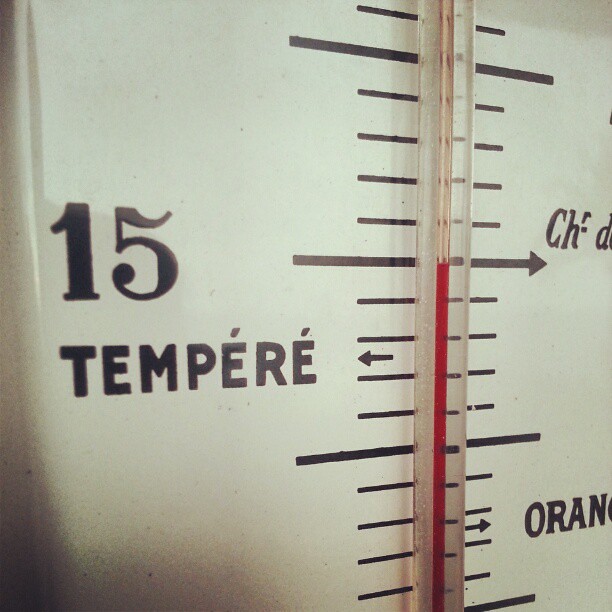This close-up photograph captures the central section of a thermostat, featuring inscriptions in what appears to be a foreign language, likely Spanish or Italian. Prominently displayed is the word "Tempere," which suggests a reference to temperature. Positioned above this term is the number 15, all set against a white background with black lettering and numerals. The glass tube of the thermometer, containing a red line to indicate temperature, is securely affixed to the thermostat. This red line aligns with the 15 mark, although the specific scale—whether Celsius or another—remains unclear. On the right side of the thermostat, partially obscured text includes the letters "CH-D" and the beginning of a word starting with "O-R-A-N." The photograph's tight crop limits visibility, preventing a comprehensive reading of the thermometer's temperature.